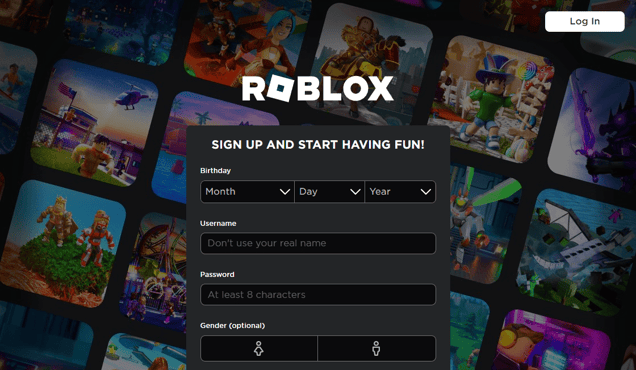**Roblox Sign-In Screen Description**

The screenshot presents the Roblox sign-in screen, prominently featuring a dark charcoal gray box inviting users to "sign up and start having fun." The first section prompts visitors to enter their birthday with dropdown menus for the month, day, and year, all set against a black background with accompanying arrows for selection.

Below the birthday input, the username field subtly advises, in gray text, against using one's real name. The next field, for the password, specifies a requirement of at least 8 characters. An optional gender selection follows, offering male and female icons to choose from.

Dominating the top center of the page, the recognizable Roblox logo is displayed in blocky text; notably, the first 'O' is designed as a square. In the top right corner, a login button is available for users who already have existing accounts.

The background of the screen exhibits a pattern of repeating, rounded squares, each showcasing various pictures related to activities, games, and characters within Roblox. These squares, reminiscent of Lego themes, are dimmed to emphasize the sign-up box in the foreground. Within these images, characters are depicted engaged in dynamic actions such as running from a helicopter, jumping out of bushes, and participating in fantastical scenarios involving dragons and other imaginary elements.